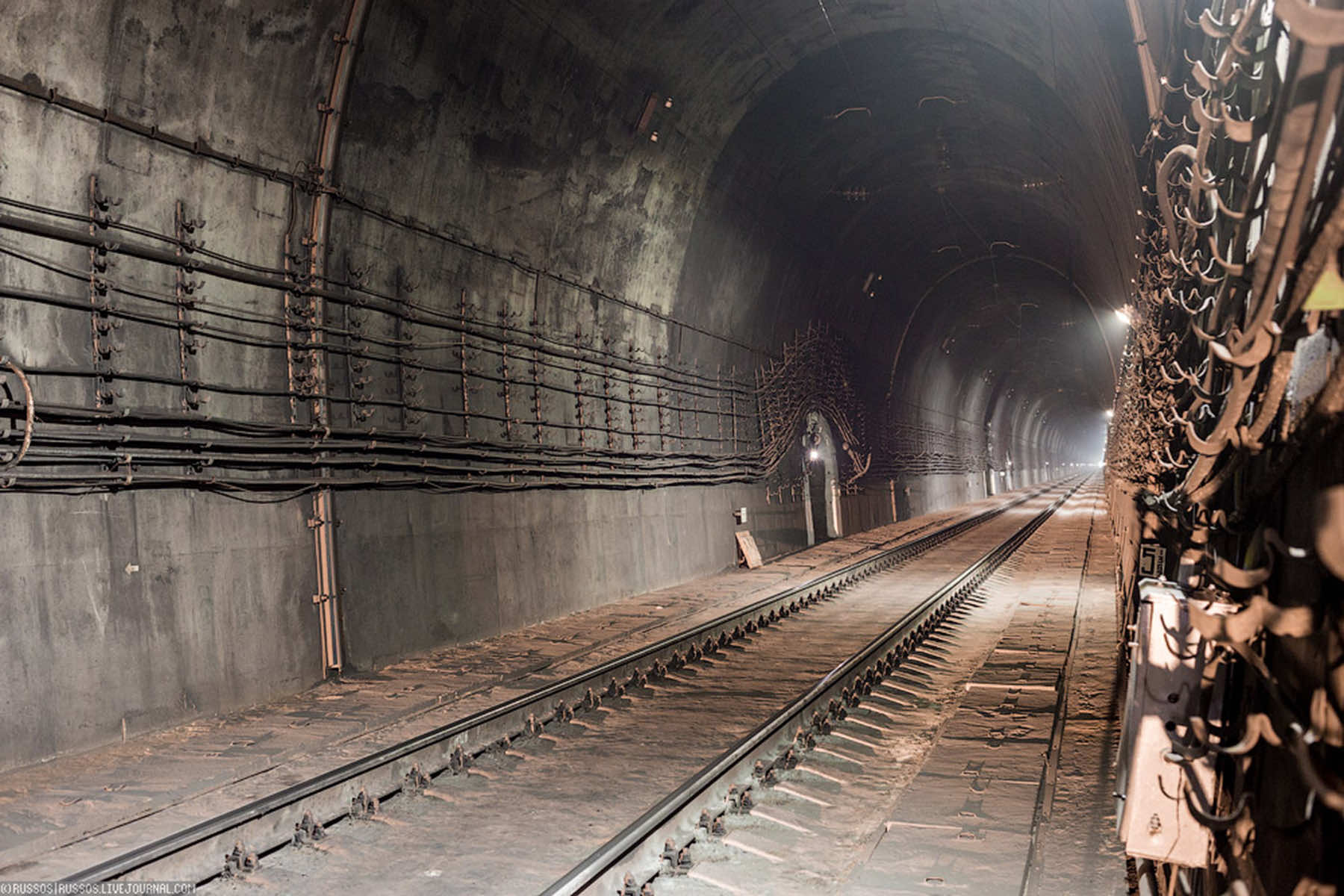This image showcases a relatively clean and well-lit underground subway tunnel, possibly in an East Coast city such as New York. The tunnel, which has a single railway track running along the center, is devoid of any trains, suggesting it might be under maintenance. The walls are predominantly gray with darker patches and are lined with intricate cables and pipes running along the length of the tunnel. On the left side, there are metallic cables and a door with a light above it, with cables curving around the door and continuing along the wall. On the right side, various metal hooks and a utility box can be seen. The ground appears dusty, and although the tunnel looks old with visible stains and watermarks, it is relatively well-maintained, free of trash or debris.